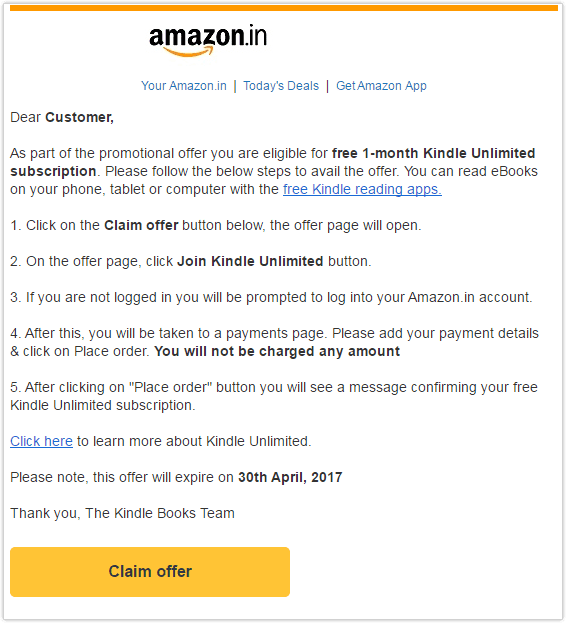This image is a screenshot of a promotional message from Amazon.in. It features a very thin gray border around it and a slightly thicker orange border at the top. Approximately two inches from the left, in bold black text, it reads "Amazon," followed by "IN" beneath it. An orange arrow, similar to the one seen on Amazon trucks, extends from the left, swooping down and then upwards.

Below this, in blue text and smaller font, it states, "Your Amazon.in." A vertical black line divides the sections "Today's Deals" and "Get Amazon App," which are placed beside each other.

On the left side of the message, it starts with "Dear Customer," followed by a body of text explaining the promotional offer: "As part of a promotional offer, you are eligible for a one-month free Kindle Unlimited subscription. Please follow the steps below to avail the offer. You can read ebooks on your phone, tablet, or computer with," followed by a blue, underlined link stating "Free Kindle Reading Apps."

The steps to claim the offer are listed as follows:
1. "Click on the 'Claim Offer' button below. The offer page will open."
2. "On the offer page, click the 'Join Kindle Unlimited' button."
3. Instructions about "Your Amazon account."
4. Information regarding the "Payment."
5. Steps for "Clicking 'Place your order.'"

Further, a blue, underlined link says "Click here to learn more about Kindle Unlimited," accompanied by the offer's expiration date. The message concludes with "Thank you, the Kindle Books Team."

At the bottom of the message, there is a large orange tab with black text indicating, "Claim Offer."